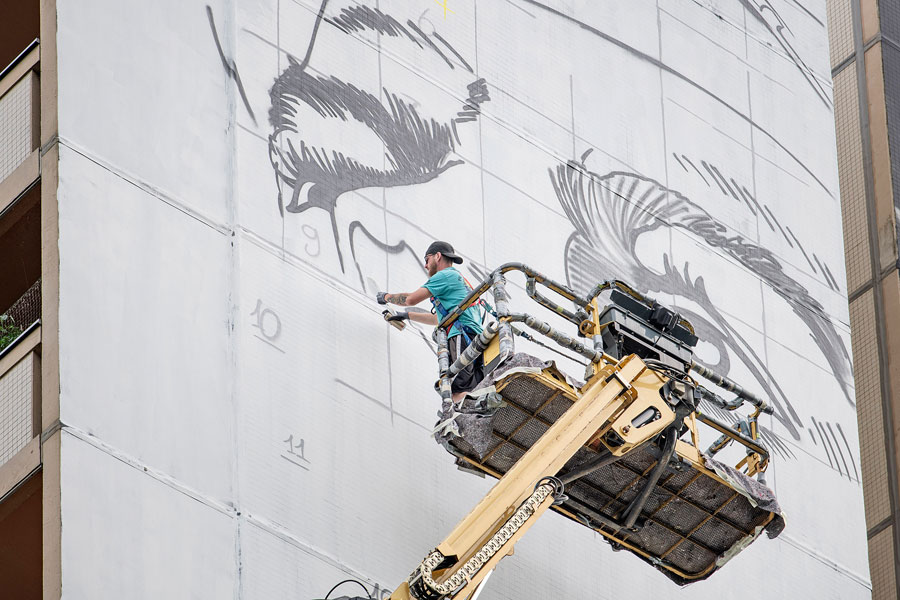In this vibrant landscape photograph, a man in his 20s or 30s, adorned in a backwards black baseball cap, light blue t-shirt, and shorts, is intently working high above the ground on a cherry picker forklift. His forearms, marked with tattoos, reveal his dedication as he deftly spray paints a large-scale mural on the side of a towering building. The artwork, which appears to be in its nascent stage, features grid lines aiding the intricate design. The mural depicts the face of a woman, with her eyes, eyelashes, eyebrows, and part of her nose already taking shape. The man concentrates on adding details to the nose as he brings the vision to life. The immensity of the wall art project suggests it will take considerable time to complete, leaving observers eager to see the finished piece.